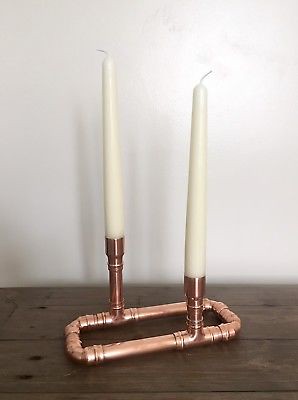The image depicts an unusually engineered candelabra made from copper or brass-colored metal tubes. The candelabra features a horizontal rectangular base formed by four tubes connected at the corners with gentle curves, resembling copper plumbing pipes. From this flat, dark wooden surface-mounted base, two additional tubes extend vertically to hold the candles. These candleholders are asymmetrically positioned at opposite sides of the rectangle, with one tube slightly taller and staggered. The two tall, white tapered candles inserted into the vertical tubes are brand new, with their wicks unlit and protruding from the top. The background consists of a plain white wall, highlighting the distinctive design and craftsmanship of the candelabra.